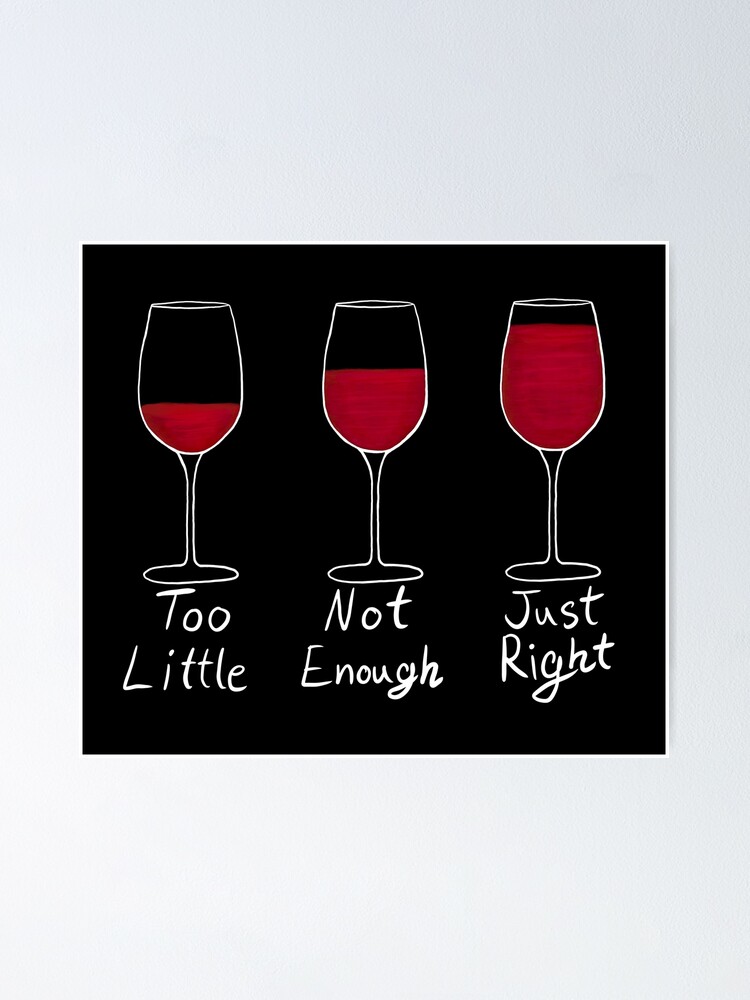This is a modern art poster that features three sketched wine glasses, outlined in white against a black background. The poster, which is mounted on a light gray wall, is framed so narrowly that the frame appears only as a thin white line. Each wine glass illustration includes a corresponding humorous label in a comic font: the glass on the left is filled one-third of the way up and labeled "too little," the middle glass is filled slightly over halfway and labeled "not enough," and the rightmost glass is nearly filled to the brim, labeled "just right." The red wine levels in each glass visualize the varying satisfaction from too little to just right, making this artwork an amusing commentary for wine enthusiasts.